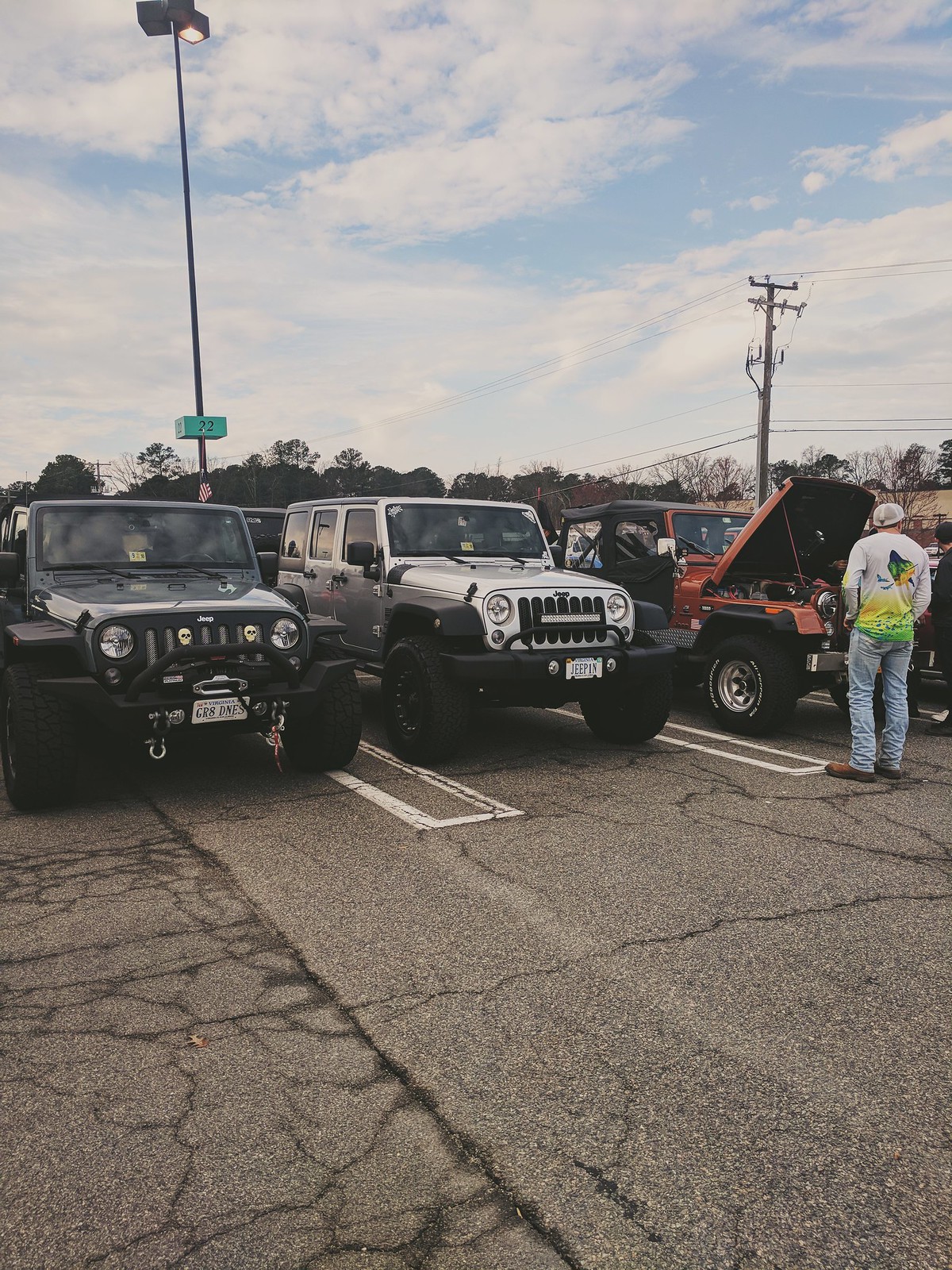This detailed outdoor photograph captures an auto show in a parking lot, showcasing three pristine Jeep Wagoneers arranged from left to right. The leftmost Jeep is black, featuring Jeep's signature vertical grille, circular headlights, and a license plate reading "GR8DNES." Next, in the middle, is a silver Jeep with black mudguards, black bumper, and wheels, complemented by an LED light bar on its rollover bar; its license plate reads "JEEP IN." Finally, on the right stands a burnt orange Jeep with black doors, back doors, and roof, its hood open as a man in a white baseball cap, white long-sleeved shirt with green and yellow designs, light jeans, and brown work boots inspects the engine. The parking lot's gray asphalt, marked with white lines, extends in the foreground under a partly cloudy sky. An American flag and a pole numbered 22 can be seen in the distance. Together, these elements beautifully set the scene of a Jeep enthusiasts' gathering.